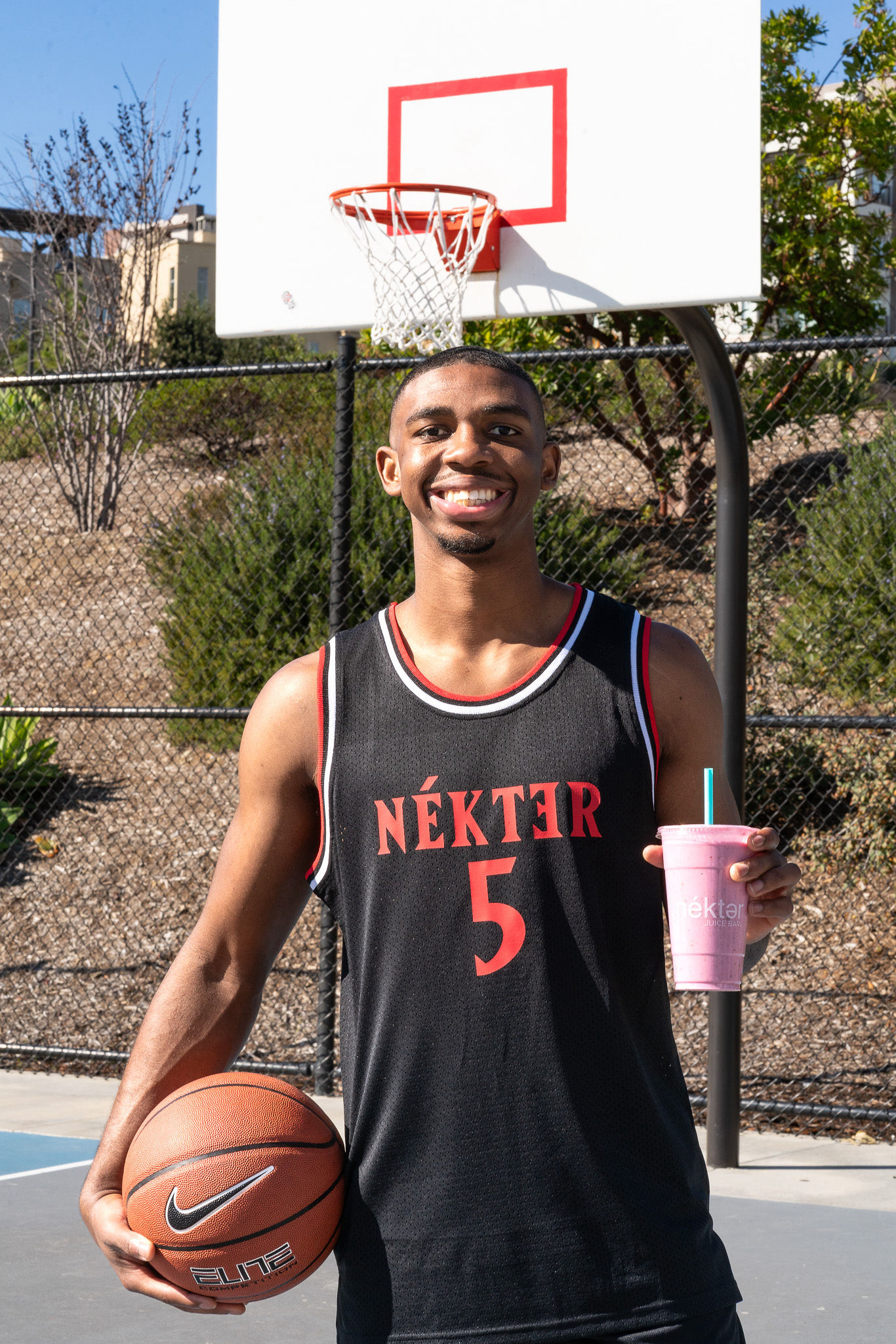In this outdoor daytime photograph, a young man of African descent stands on a basketball court, smiling broadly at the camera. He has very short black hair, a mustache, and a sole patch on his chin, giving his round face a cheerful appearance. The man strikes a casual pose, with his right arm extended downward, holding a basketball with the Nike swoosh logo resting against his hip. In his left hand, he holds a plastic cup containing a pink shake or smoothie, the drink's green straw adding a pop of color.

The man wears a distinctive black basketball jersey adorned with red and white stripes around the collar and sleeves. Across the chest, bold red print spells out "N-E-K-T-E-R," with an asterisk above the first "E" and the second "E" being mirrored. Below the lettering, the number "5" stands out prominently. Behind him, a white basketball backboard with an orange target square is visible, mounted on a fence. Beyond the fence, a hill with bushes adds depth to the background, completing the setting for this vibrant, personality-filled snapshot.